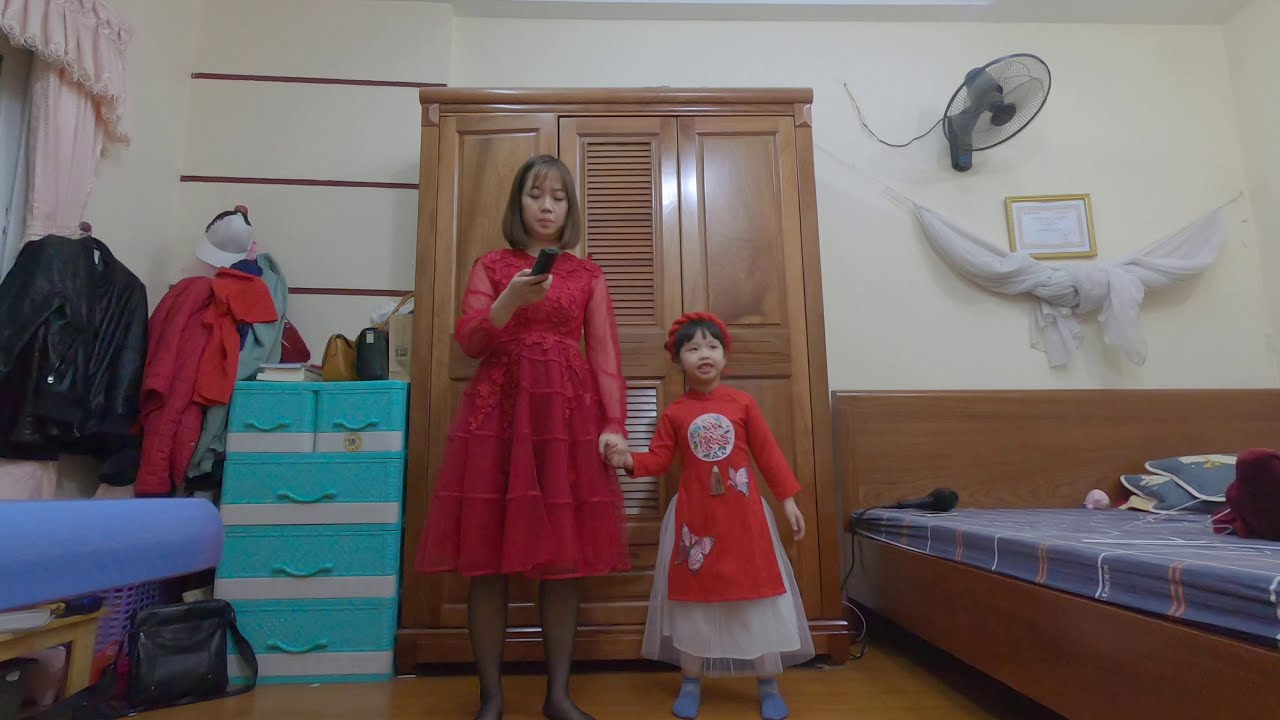In this detailed photograph, a young woman and a child are standing at the center of a bedroom, both facing the camera and holding hands. The young woman, standing on the left, is dressed in an elegant knee-length red gown with long sleeves made of layered chiffon adorned with floral designs. She holds a remote control or some kind of electronic device in her free hand. Beside her on the right, the little girl is dressed in a charming red dress with a white skirt underneath, a red top resembling an apron, and red shoes. Her hair is styled in an updo with a red ribbon tied around it. 

In the background, there is a brown armoire directly behind them and a wooden bed to the right, featuring blue sheets, pillows, and a black fan positioned above it. On the left side of the image, blue or turquoise shelves with several large and small drawers are visible, along with assorted clothing items, including jackets and yoga mats, indicating storage that might be typically found in a closet. Additionally, there's a window with curtains to the left. The room is filled with various colors including red, blue, brown, white, and gray, creating a personal and cozy indoor setting.